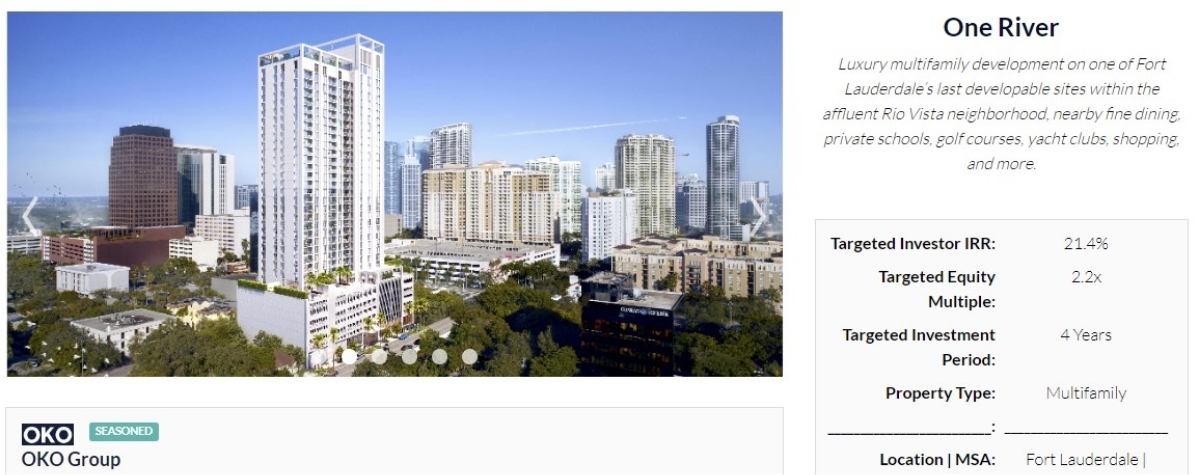Screenshot of the "One River" Luxury Multifamily Development Website:

This screenshot showcases the promotional material for the "One River" luxury multifamily development. On the right-hand side, there's a section of text set against a white background, detailing the project's prime location within Fort Lauderdale's prestigious Rio Vista neighborhood. The description highlights its proximity to fine dining, private schools, golf courses, yacht clubs, shopping centers, and more.

Beneath the descriptive text, there is an investor information table. This table provides key metrics for potential investors including the targeted internal rate of return (IRR), targeted equity multiple, targeted investment period, property type, and location specifics.

To the left of this textual information is a large, landscape-oriented photograph capturing a vibrant view of Fort Lauderdale. The image depicts a clear sky above a sprawling cityscape, characterized by multiple high-rise and mid-rise apartment complexes. Dominating the center of the photo is a prominent white square apartment building, surrounded by various multi-colored apartment complexes nestled among abundant green trees.

Below this main photo, there is another element with black text on a light grayish background, indicating the involvement of OKO Group. The text reads "OKO seasoned" followed by "OKO group." The photograph above is part of a slideshow, as evidenced by navigational arrows on both sides of the image and dots at the bottom signaling multiple other photos available for viewing.